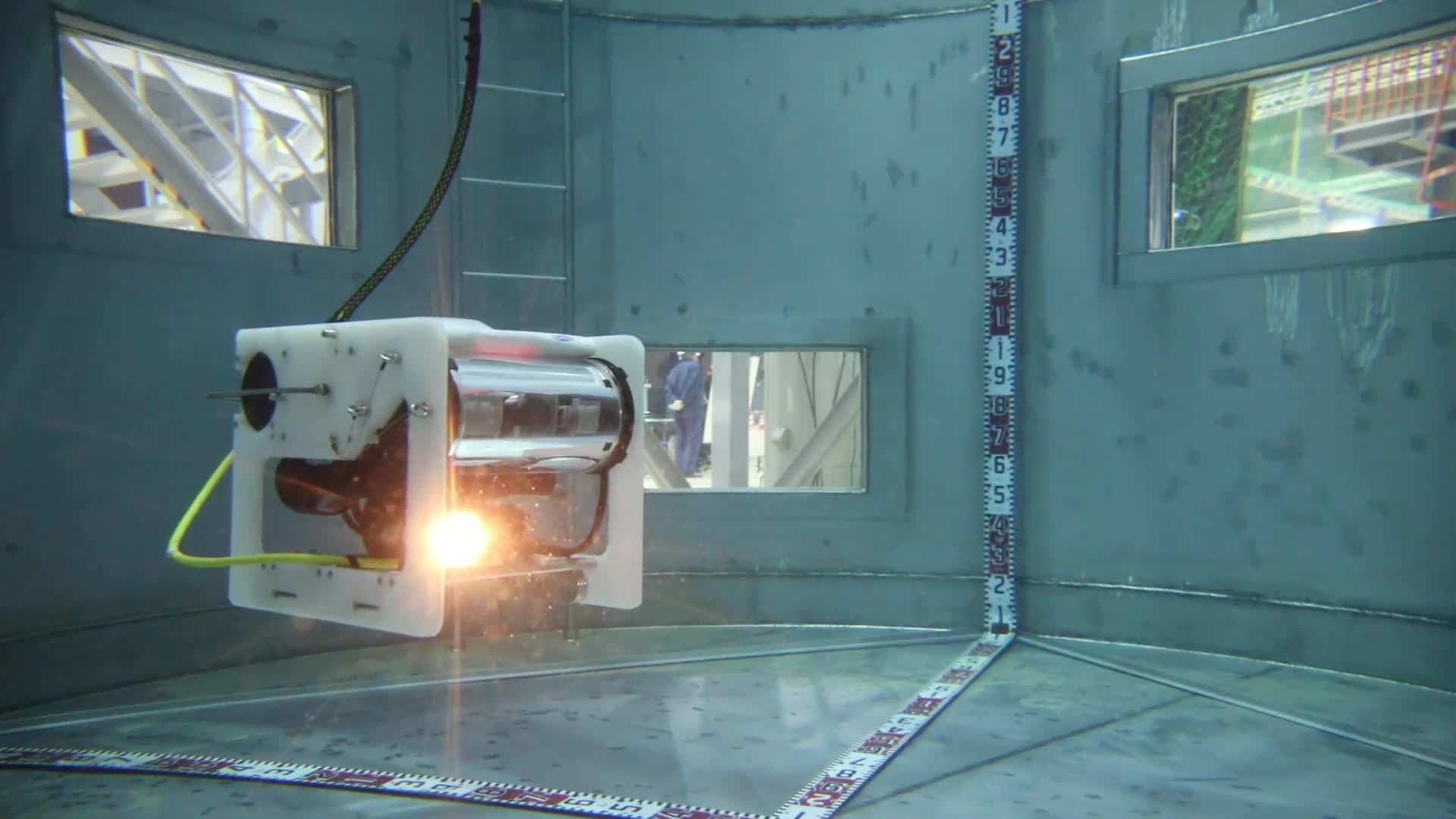The image depicts the interior of a bluish-gray, somewhat circular room that has the appearance of a scientific research tank or an advanced x-ray room. The walls are made of metal and glass with a turquoise hue, and there are three rectangular glass windows: one above the main device, one on an adjacent wall revealing a white stairwell, and another low to the floor showing steel beams and a man outside. Dominating the scene is a complex, roughly cubical machine, seemingly suspended from the ceiling by a black, snake-like metal arm. This machine features white plastic sides with metal cylinders inside, possibly resembling rollers akin to a printing press, and an intriguing bright orange light at its base. Extending from the machine is a green wire that transforms into a black cord leading out of the frame. Below, two metallic strips radiate across the floor from the center, marking out a pie-shaped section of the room. Adjacent to these, a red and white measuring tape with numerical markings extends along the floor and wall, adding to the overall precision-focused and technical ambiance of the space.